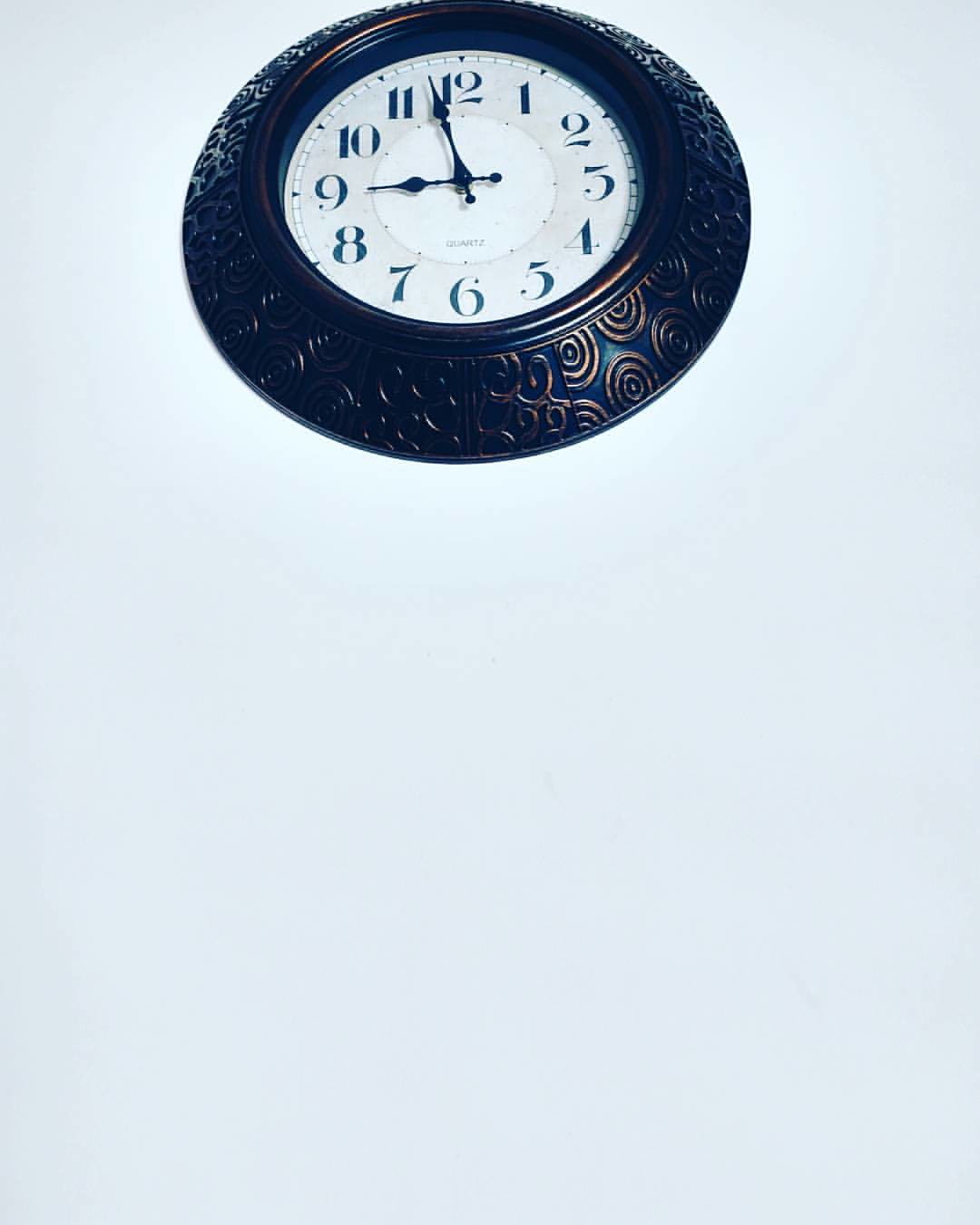In this photograph with a light blue background, a wall clock prominently occupies the upper center of the image. The clock is round with a metal frame that combines dark blue or black with intricate bronze detailing. These decorations consist of concentric circles and swirling, vine-like patterns. The face of the clock is white, featuring black numbers from 1 to 12 and black hands pointing to 8:58. A slight shine reflects off the bronze details, suggesting light from the lower right. The clock's intricate design and prominent positioning against the backdrop create a striking visual contrast.